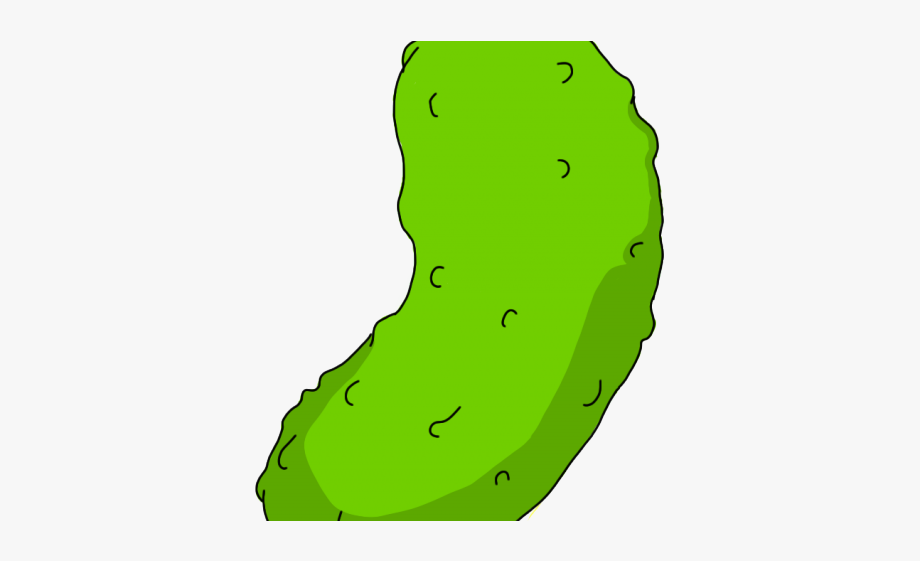The image features a digitally created, cartoon-style pickle prominently centered within a rectangular frame. The pickle, depicted in light green with a darker green base, is outlined in black and decorated with 12 black half-circle textures, giving it a spiny appearance. These textures are dispersed in a somewhat irregular pattern along its surface. The composition has a simple background that is predominantly light gray, though it appears slightly lighter in the upper left-hand corner. The pickle is oriented vertically and seems to be facing the right, with its bulkier end on the right side. There are no additional elements or text in the image, emphasizing the pickle as the sole focal point against the minimalist backdrop.